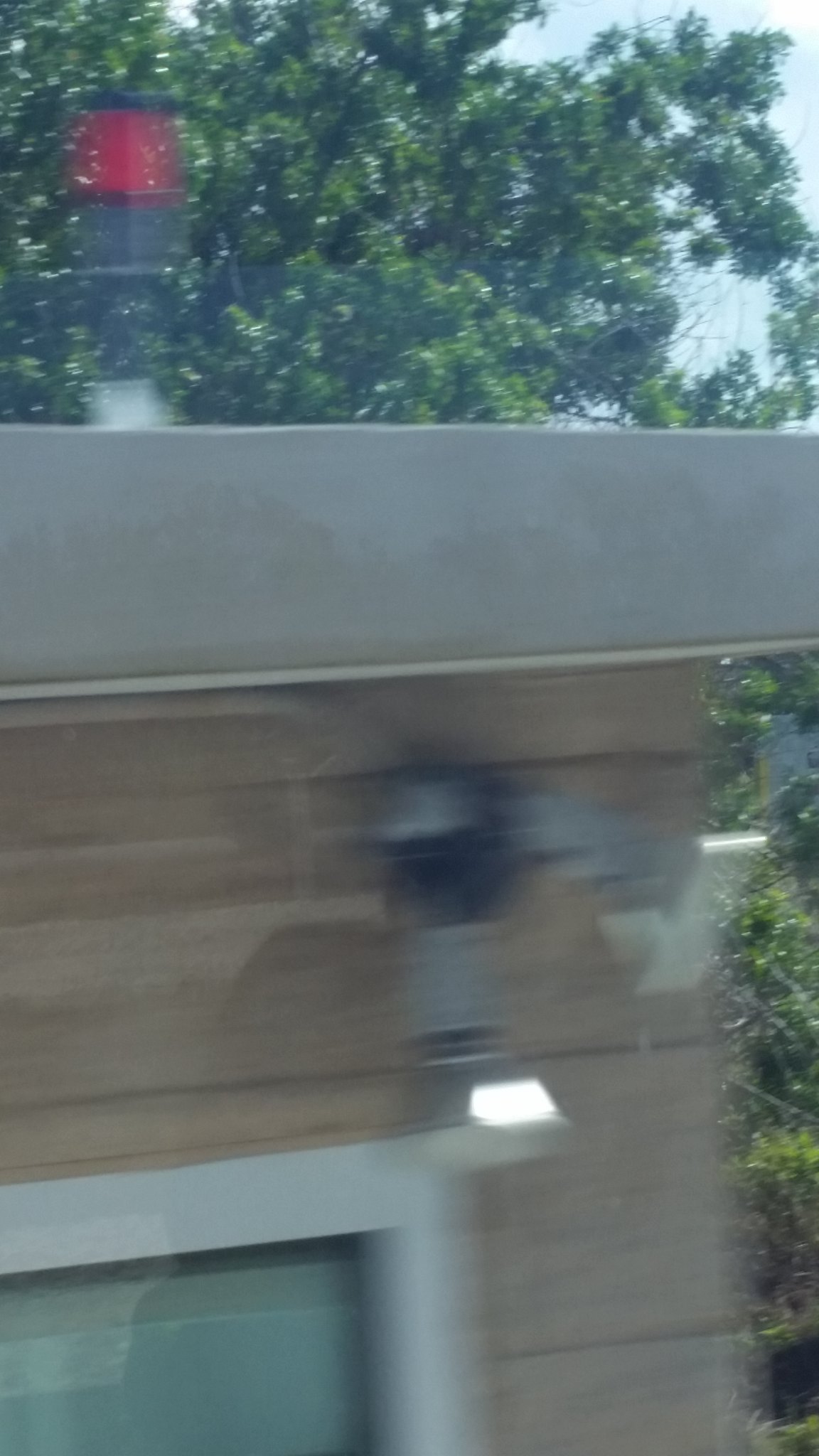The image depicts a blurry photo of the side of a beige, one-story house with a flat, light gray roof. A distinct red-topped cylindrical structure, possibly a chimney or emergency light, is visible on the roof. The house's exterior features wide, horizontal wood paneling, and at the bottom left corner, part of a window with white trim is visible. Attached to the wall near the top right of the building is a floodlight, and possibly another device like a security camera. Green, fluffy trees with a blue sky peeking through their leaves form the background, adding a natural contrast to the man-made structures. The overall blur of the photo and reflections, especially toward the bottom left, suggest it was likely taken through a window, making it challenging to discern all the details clearly.